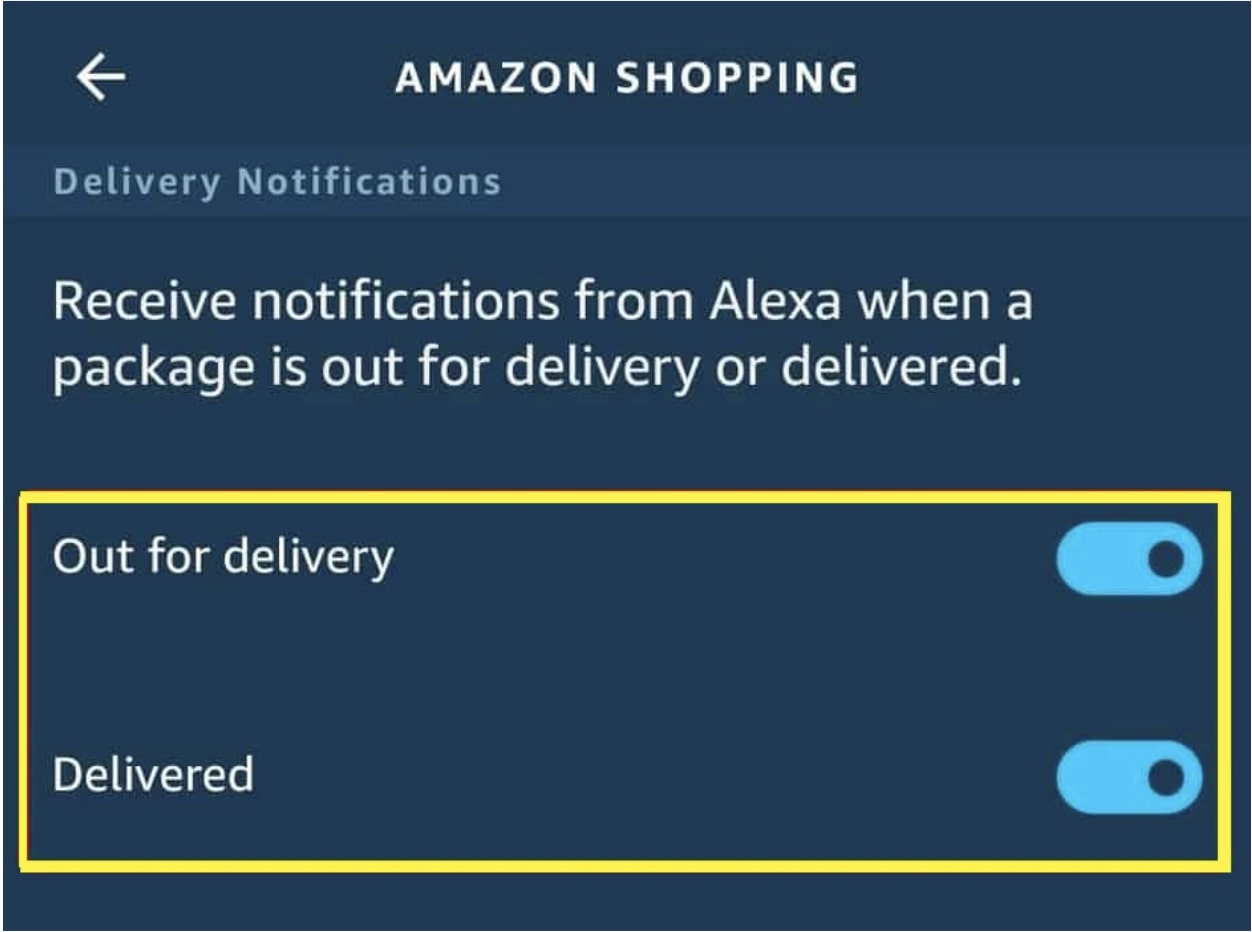The image is a screenshot captured from the Amazon website, featuring a dark gray background. In the upper left corner, a white arrow points to the left. To the right of this arrow, the text "Amazon Shopping" is displayed in bold white font. Just below, a narrow gray banner stretches across the screen, containing the light blue text "Delivery notifications." Beneath this banner, the text "Receive notifications from Alexa when a package is out for delivery or delivered" appears in white. Below that description is a yellow bordered box with the text "Out for delivery," accompanied by a blue toggle button to the right, indicating that the toggle is switched on. Further below, the text "Delivered" is displayed, also with a blue toggle button to its right, which is similarly turned on.